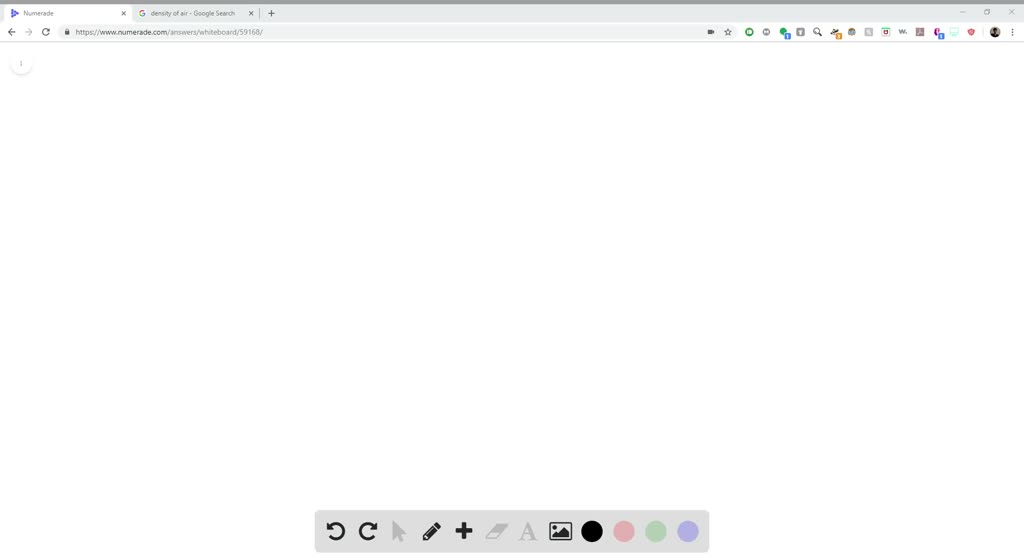Screenshot of a website interface, featuring a gray toolbar at the top. The toolbar includes icons for reverse (undo) and redo actions, both in a faded style, along with a pencil and eraser, the latter also shaded. There's a faded letter "A" and a portrait icon. Four colored circles—black, pink, green, and a purplish-blue—are visible. Two tabs are open at the top, and the website's address is displayed. In the top-left corner, there's a white circle with two gray dots. In the top-right corner, there's a dash, two overlapping squares, and an "X." Also in this corner is a profile picture next to three vertical dots. The search bar displays a lock icon before the website address. On the right side of the toolbar, there's a black rectangle with a star.